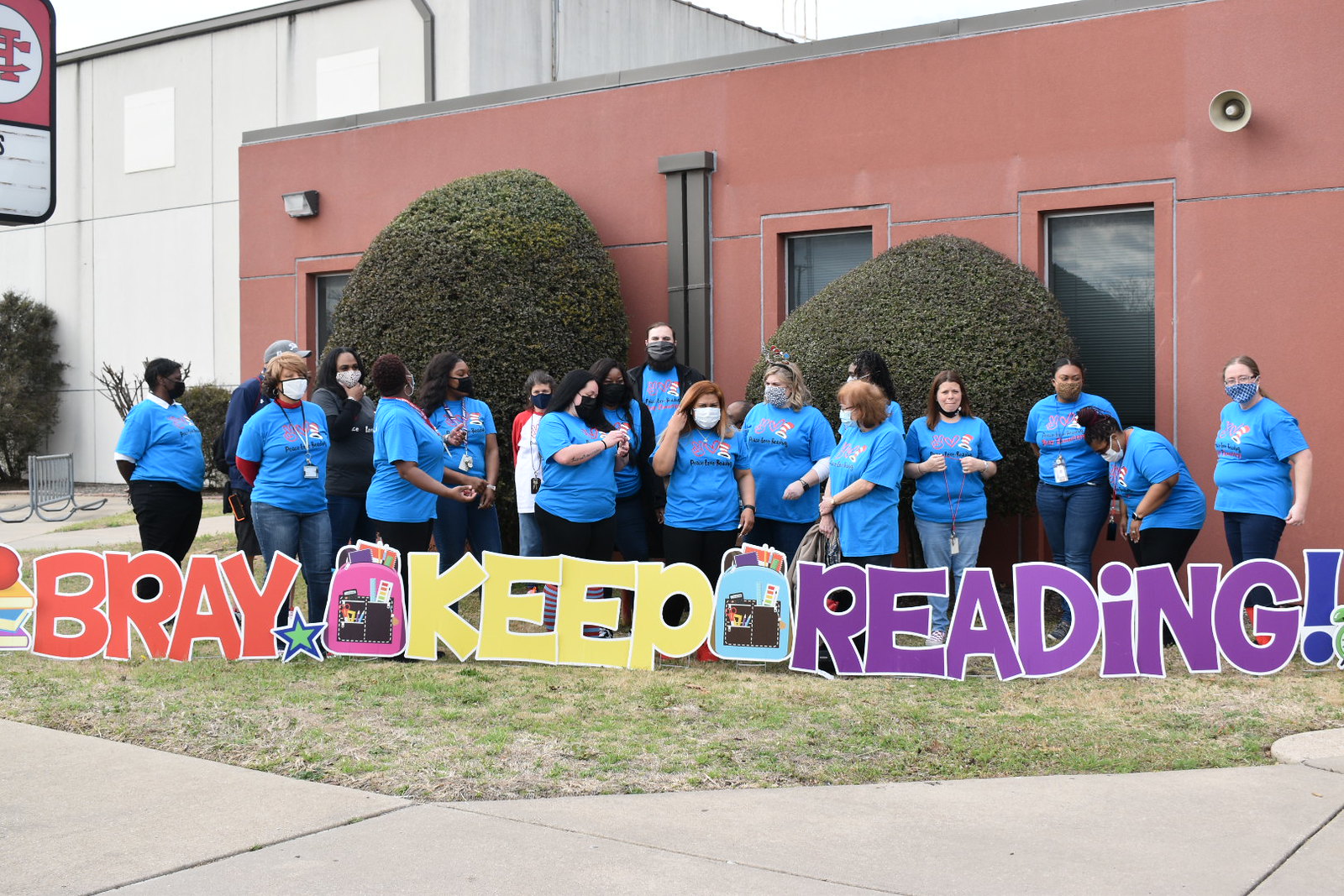A group of people, likely educators or library staff, are standing outside in front of a red stucco building with two large, rounded green bushes in front of it. The building is a single-story structure with three visible windows and a well-maintained sidewalk at the lower part of the image. The group, predominantly women, is uniformly dressed in light blue t-shirts featuring a design that isn't entirely clear, paired with blue jeans or dark pants. Most of them are wearing face masks. Superimposed across the lower portion of the photograph are cut-out letters spelling "keep reading" in colorful letters, with 'Bray' in orange followed by a yellow backpack, another backpack, and "reading" in purple with a blue exclamation point. Some individuals in the group are looking directly at the camera, while others are gazing off to the side or downward. In the background, a white building is visible next to the red one. The group is standing on a patch of grass, adding a vibrant green to the scene.